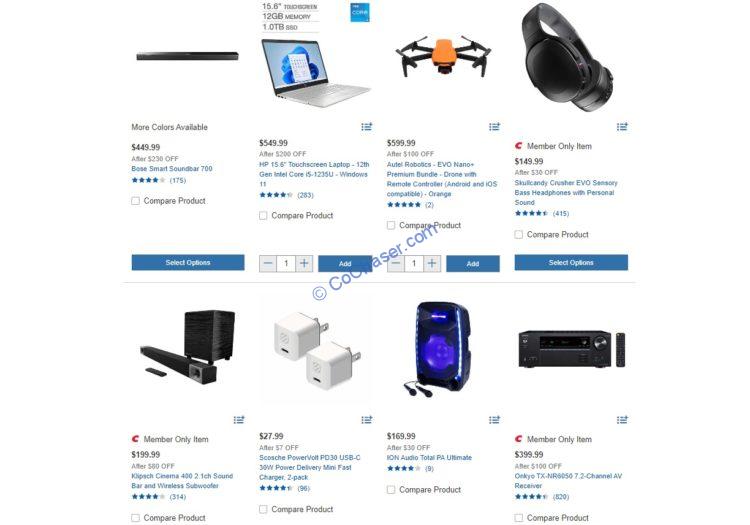This image is a detailed screenshot of the CoChaser.com webpage, as indicated by the diagonal light blue watermark with a copyright symbol. The screen displays eight items for sale, each with a description, price, and clickable link for adding to the cart or viewing reviews.

### Top Row:
1. **Bose Smart Soundbar 700** - A sleek black soundbar priced at $799. It features high-quality sound and modern aesthetics.
2. **Silver Laptop** - Priced at $549.99, this open silver laptop is detailed with multiple attributes, including processing power and storage capacity.
3. **Orange and Black Drone** - Listed at $599.99, this drone stands out with its vibrant color and features.
4. **Skullcandy Crusher EVO Sensory Bass Headphones** - A member-only item priced at $149.99, these headphones are known for their personal sound customization and enhanced bass.

### Bottom Row:
1. **Speaker Set with Soundbar** - This item includes a soundbar and accompanying speakers, designed for immersive audio experiences.
2. **Plug-in Chargers** - Simple, wall plug-in chargers, ideal for various electronic devices.
3. **Speaker** - Another speaker option, detailed with specific audio features.
4. **Stereo Receiver System** - A comprehensive stereo receiver with all necessary attributes listed, aimed at enhancing home audio systems.

Each product entry is accompanied by clickable links for more detailed reviews or to add the item to the shopping cart.